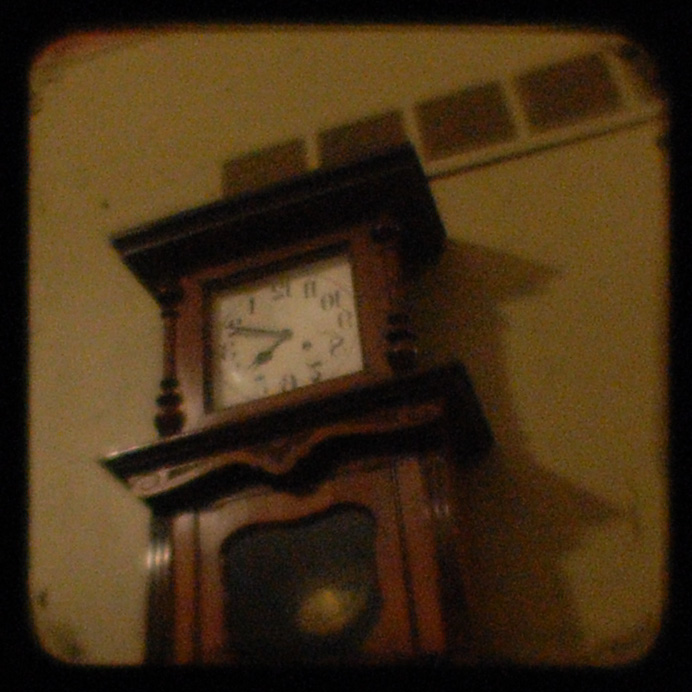This image showcases a vintage grandfather clock, characterized by its imposing, rectangular wooden frame. The clock face, a prominent square, features a distinctive brown background outlined in black. The black numerals appear intriguingly reversed, adding an element of mystery to its historical charm. Both the long and short clock hands end in pointed tips, clearly delineating the time. The clock rests against a light brown painted wall, with its shadow casting a compelling presence on the right side. Visible through a glass pane at the lower section of the clock is a metal pendulum, accentuating the clock's mechanical elegance as it sways gently from side to side.